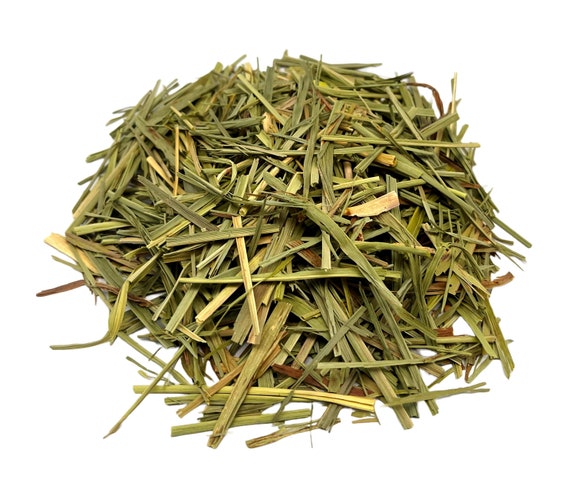The image depicts a pile of dry grass clippings, arranged haphazardly in a circular shape. The blades of grass, varying in hues from light green to brown and yellow, indicate they might have been mowed from a lawn, possibly including shaded or dying sections. The pile, roughly eight inches in diameter and about an inch or two high, is photographed from an angle, likely around 45 degrees from above. The grass, some blades being the length of a cigar, sits on a plain white background, emphasizing the contrast in colors and textures without any distracting elements. This composition suggests that the clippings have been casually gathered at the center of the image.